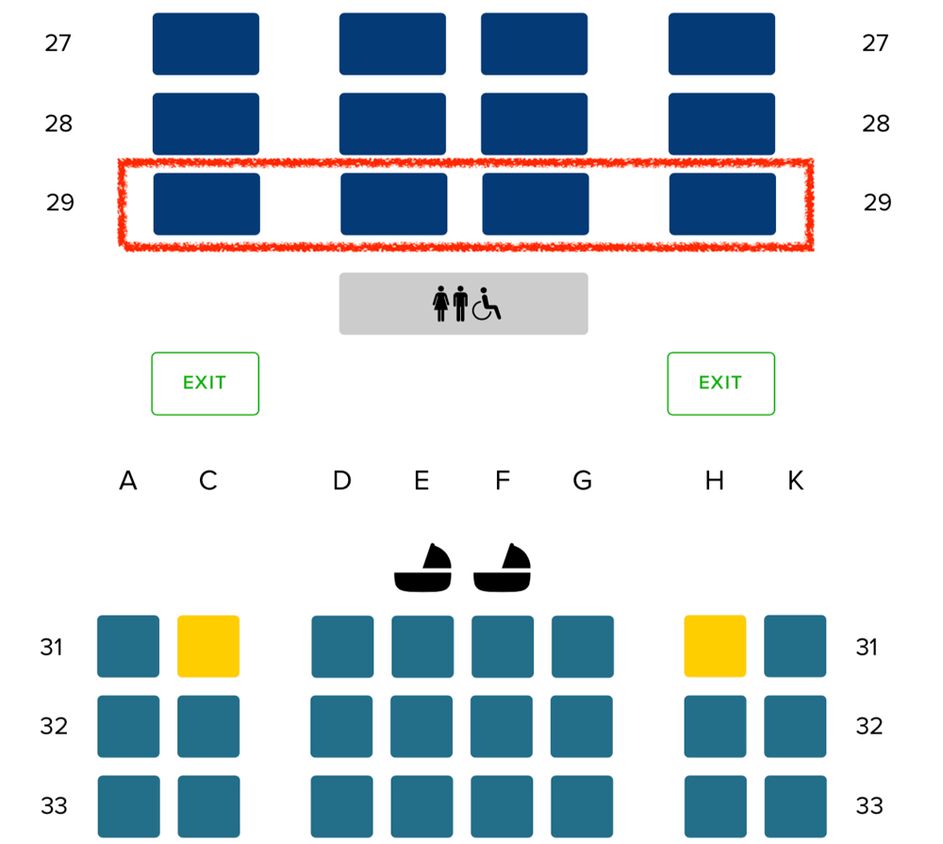This image is a detailed seating chart of an airplane, presumably from an airline's booking or information system. The chart prominently displays rows 27, 28, 29, 31, 32, and 33. There is a noticeable gap between rows 29 and 31, indicating a section break or additional facilities in that area.

Rows 27, 28, and 29 are highlighted within a red rectangular box. Each of these rows features blue rectangles that likely represent available seats. In these rows, the seating pattern shows two seats spaced apart on the outer edges (left and right) and two seats placed closer together in the middle. 

A significant gap is evident after row 29, which accommodates restrooms in the center, marked with gray icons depicting a man, woman, and a wheelchair, suggesting accessibility features. Following the restroom area, the exits are indicated on both the left and right sides of the aisle.

Continuing with the seating chart, rows 31, 32, and 33 follow after the gap. The columns for these rows are labeled A, C, D, E, F, G, H, and K, spanning across the chart.